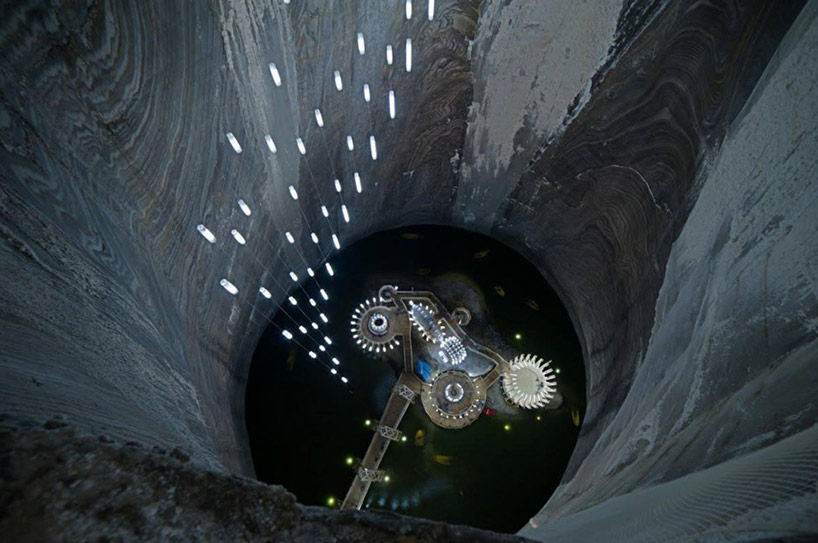The image depicts a cavernous, tunnel-like environment, probably an animated or concept art scene, which suggests a video game setting. The scene features a dark, man-made, circular hole with rocky, striated walls, transitioning from light gray at the top to deep black as it descends. In the center of the image, a glowing motorcycle, seemingly part of the animation, traverses a platform illuminated by green lights. This platform, appearing as an assemblage of cogs or gears, has walkways with lights that connect different parts. Dangling from above are thin, cylindrical lights, adding to the otherworldly ambiance. Far in the background, a white, fan-like structure emerges, enhancing the intricate detail of the scene.